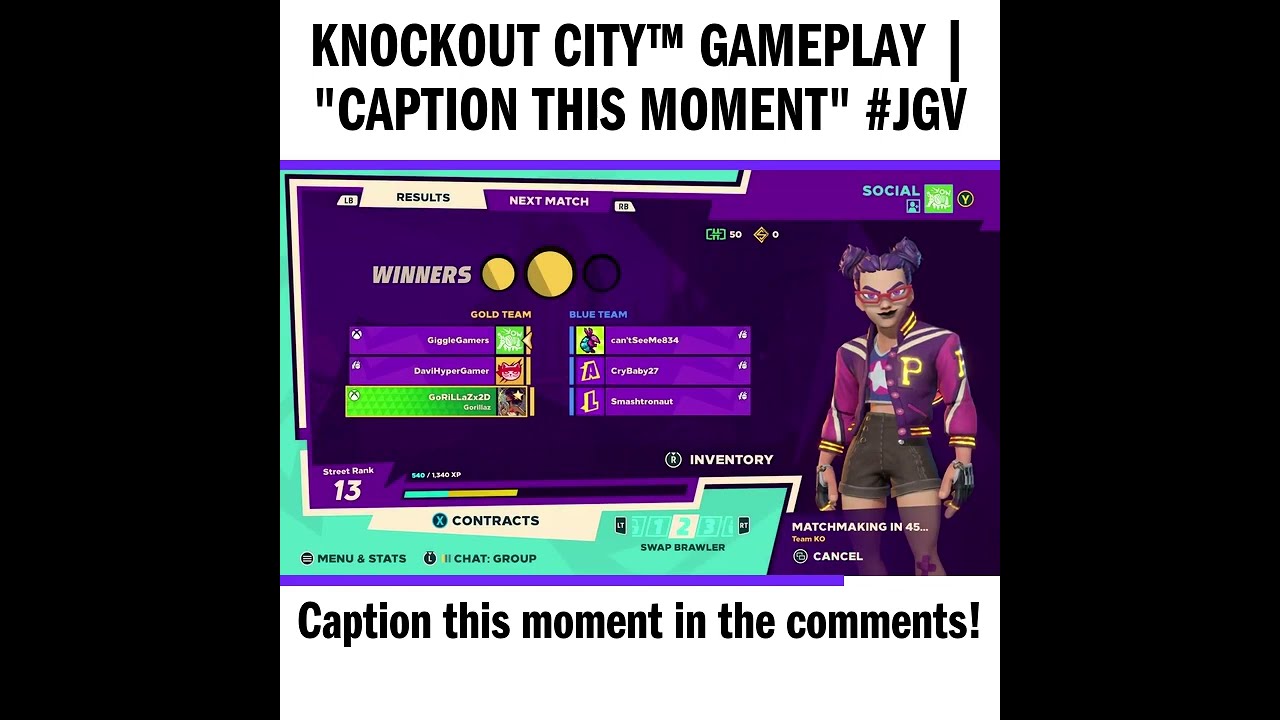The image is a digital screenshot from the video game Knockout City™ with a clear layout meant for prompting comments. It features a predominantly blue and purple color scheme with accents of neon green and yellow. Two white bars frame the image at the top and bottom, housing black text. The top bar reads, "Knockout City™ Gameplay - Caption this moment" followed by hashtag JGV, while the bottom bar instructs, "Caption this moment in the comments!"

The central part of the image contains a vivid depiction of a game character set against a black background. This character, a girl with brown hair in pigtails, sports red-rimmed glasses and a purple and yellow varsity-style jacket with a letter 'P' over the chest. She also wears khaki shorts. To her left is the leaderboard, highlighted with neon purple and teal blue borders. The leaderboard features the word 'Winners' in gold above two yellow globes, and details two columns of three entries each. The left column's last entry is highlighted in neon green, indicating the player who took the screenshot. The right column lists players with icon images next to their names, such as 'Crybaby27.'

Below the character, the image has a teal-blue border with a white horizontal bar reading "Contracts" in black lettering. There's additional small, mostly unreadable text over the teal border and a transparent black box over the character's legs with white text and a visible "Cancel" at the bottom row. The overall aesthetic reflects a vibrant, competitive environment complete with detailed visual elements and virtual sport-like attire.